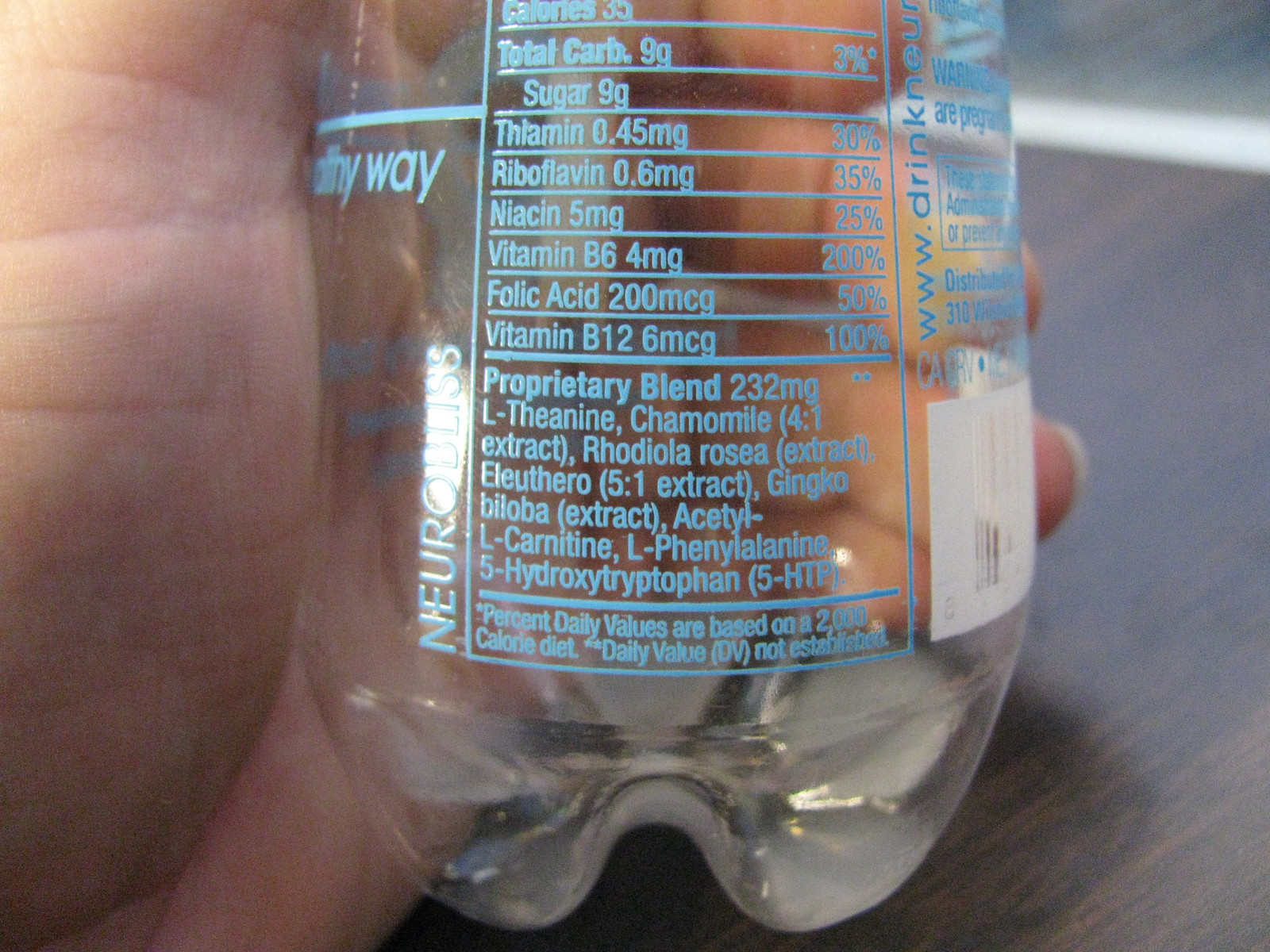The image depicts the bottom half of a clear plastic bottle, likely containing a nutritional water or energy drink. The bottle is held in someone's left hand, resting on a dark wood-grained table. The label, printed in light blue ink, highlights the nutritional facts, including 9 grams of sugar, 6 milligrams of riboflavin, and a proprietary blend of 232 milligrams containing ingredients like L-theanine, chamomile extract, L-phenylalanine, and 5-hydroxytryptophan. The label also lists vitamins such as thiamin and folic acid. Some text on the label appears slightly blurry, and there is a small white strip at the bottom of the bottle. The person holding the bottle has white skin and faint white nails. Only the bottom half of the bottle is visible, with the contents just below the nutrition label. The text "NeuroBliss" runs vertically along the left-hand side, and a barcode is located near the bottom right of the label.